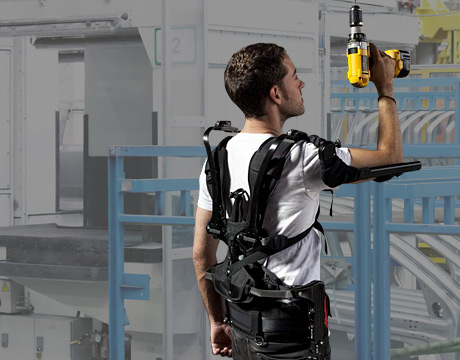The photograph captures a young man with fairly pale skin, dark brown hair, and stubble around his jaw and chin, standing at an angle with the side of his head visible. He is wearing black pants and a white short-sleeved t-shirt. Strapped to his back is a black exoskeleton device designed to aid in lifting, which attaches around his back and extends across his arms, with visible connections at his elbows. In his right hand, he holds a yellow, silver, and black powered drill, pointed upwards as if he is focusing intently on a task above him. The backdrop features a bluish-white metallic setting with elements like steel beams, the side of a ship, and an elevator, creating the impression of an industrial environment, although it appears to be a staged background rather than an actual outdoor scene. The man’s serious expression underscores his concentration on the job at hand.